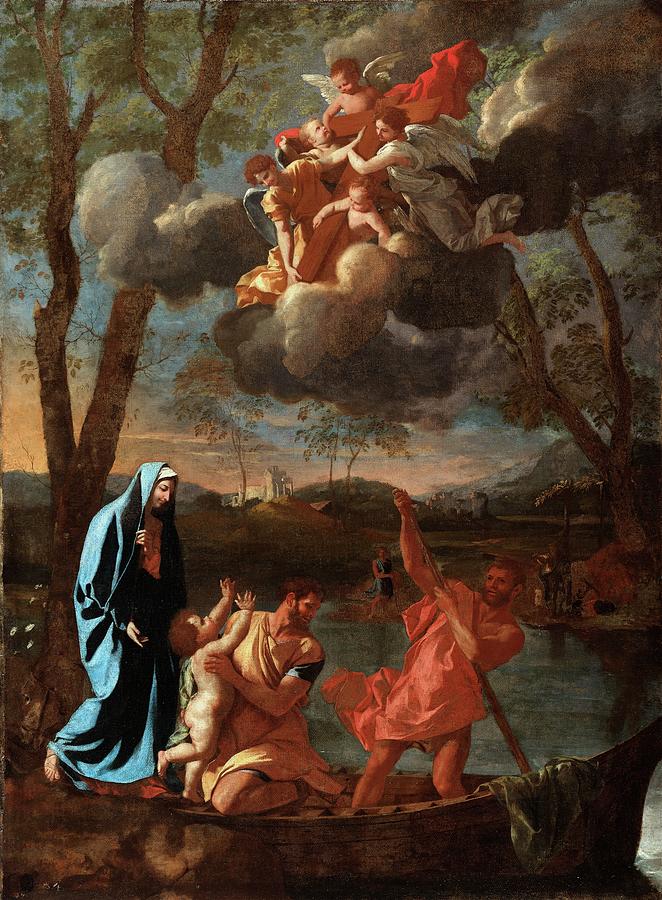This vertically aligned, rectangular painting, which appears to be several centuries old, features a small, brown canoe occupied by three adults and a chubby baby. On the right side of the canoe stands a man with short brown hair and a goatee, wearing a red or orange gown, holding an oar. In the middle is another man with similar short brown hair and a goatee, draped in a garment over one shoulder and another dark cloth around his bare shoulder, holding the baby who reaches upwards. To the left, a woman in a blue gown, reminiscent of a nun's habit, extends her hand towards the baby's head. The background depicts water with a person standing on the opposite bank, surrounded by trees with brown trunks and green leaves, under a sky filled with layers of blue, pink, and gray clouds. Above, five angels – two cherub-like children and three with wings – float among the clouds and trees, adding to the painting’s religious atmosphere. The scene captures a moment filled with divine and serene elements, resonating with spiritual symbolism.